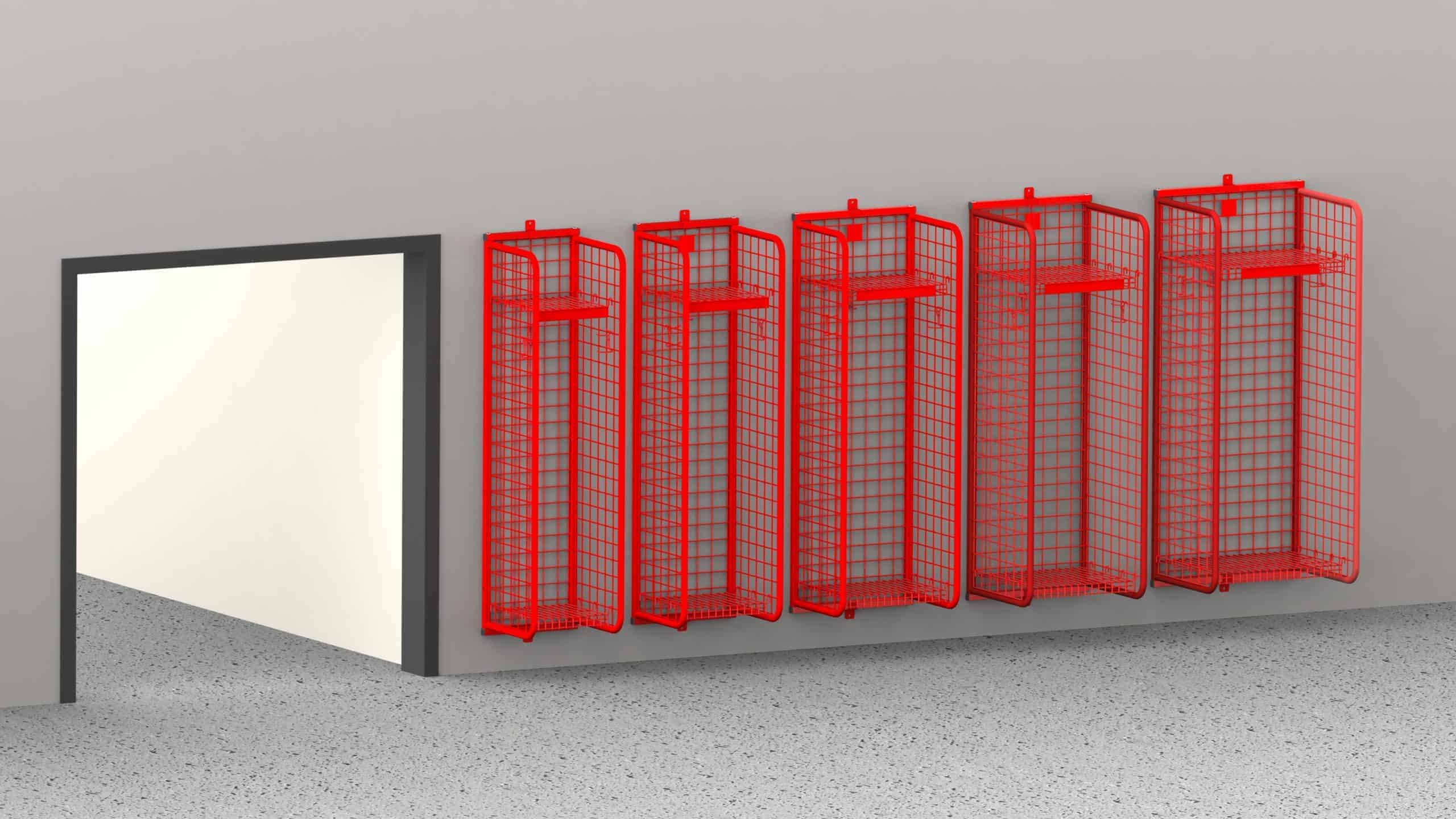The photograph captures the interior of a building featuring a large, doorless doorway on the left, framed in gray and leading to a hallway with white walls. The main room showcases a series of five red, grid-like metal racks mounted on a gray wall. Each rack, resembling a cage with three enclosed sides and an open front, increases in size from left to right, creating a climbing effect. These racks, starting slightly past the midpoint of the image, vary in width and feature a single shelf at the top. The floor throughout both the main room and the hallway is a speckled tile pattern, mixing white with black or gray specks, adding to the scene's sense of depth and perspective.